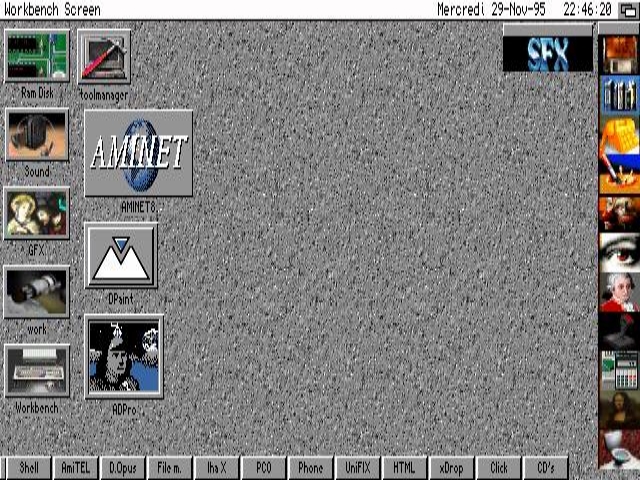The image is a screen capture of a 1990s-era computer program, depicting the "Workbench Screen" interface. Towards the top, the screen displays the date and time in black letters: "Mercredi 29 November 1995, 22:46:20." The background has a black and gray speckled texture, reminiscent of asphalt. On the left, there are icons labeled Aminet, Workbench, Work, Depaint, GFX, Sound, and Ramdisk. The top right features an icon box labeled "SFX" with a black background and blue, shiny text. Along the bottom of the screen are small gray buttons labeled Shell, Amitel, DeOpus, FileM, eHotX, PCO, Phone, UniFix, HTML, Xdrop, Click, and COs. On the right side of the screen, a column of icons includes images such as a close-up of an eye, an orange telephone, a toilet bowl, a picture of Mozart, and the Mona Lisa painting. The overall setup suggests a graphical user interface from the mid-90s, complete with various application icons and tools.